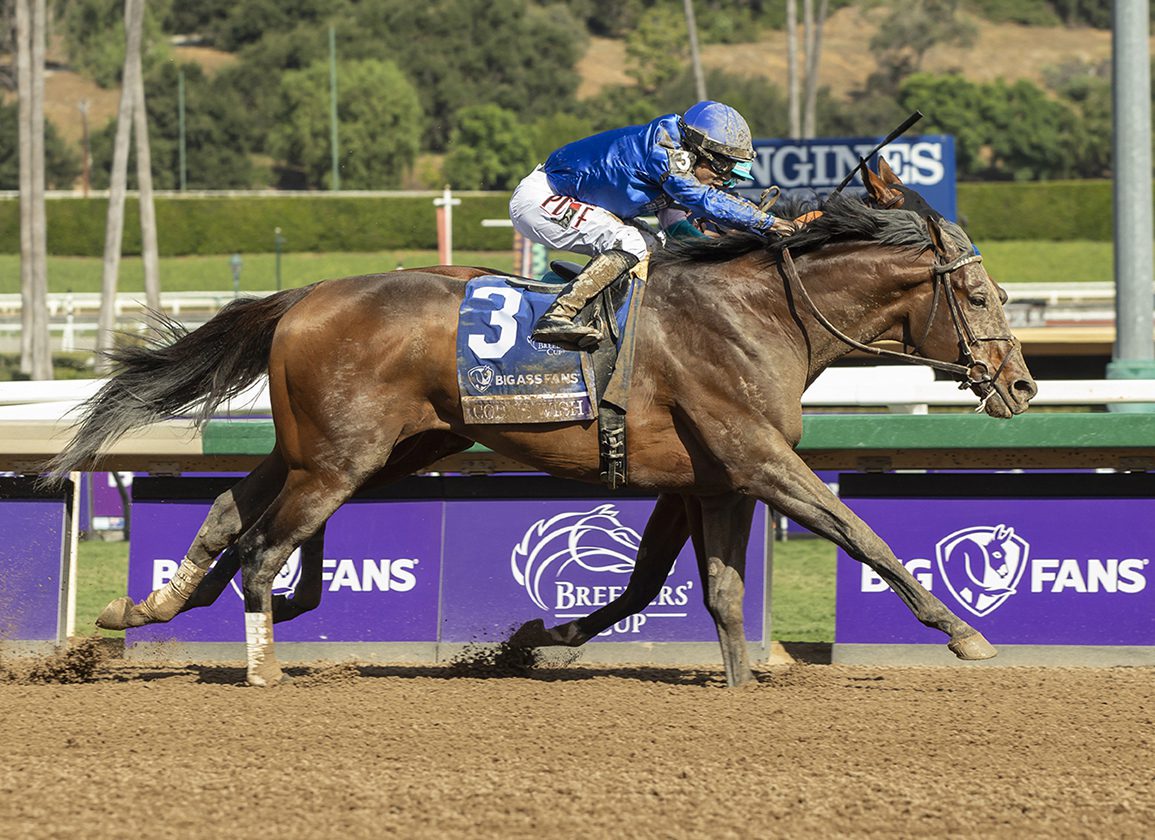This photograph captures an intense moment during a horse race, featuring a single, deep brown chestnut horse in full gallop, moving toward the right side of the frame. The horse, adorned with a blue saddle blanket emblazoned with the number three and partially obscured by mud, proudly displays the sponsorship "Big-Ass Fans". The jockey, leaning forward in a racing stance, dons a blue helmet, a matching blue jersey, and white pants, with his tall boots heavily caked in mud. The backdrop includes purple banners running along the track enclosure and additional blue banners displaying partial text "NGI" and "NES" near the jockey's head. The setting is framed by tree trunks and distant greenery, with the dirt racetrack in sharp focus beneath the flying hooves. The composition also hints at another horse racing alongside, as evidenced by visible legs peeking into the frame, adding to the dynamic racing scene.